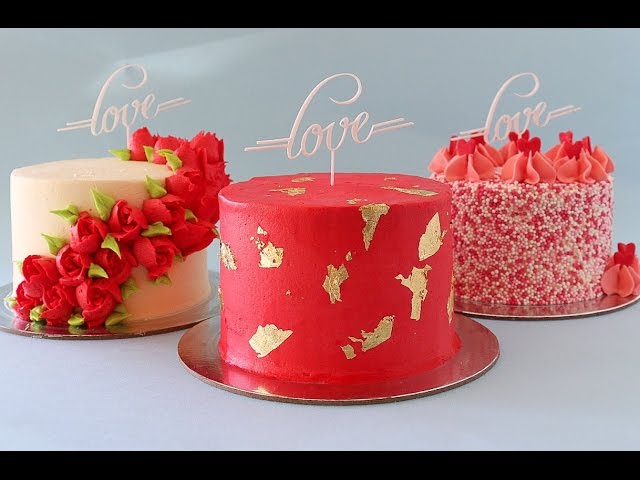This color photograph showcases three cylindrical cakes, each adorned with the word "love" written in cursive on a white plastic topper. The cakes are neatly positioned next to each other on round silver plates against a gray background. 

The cake on the left is cream-colored and elegantly decorated with red roses and green leaves encircling its surface. A delicate “love” topper is pinned to its top, adding to its romantic charm.

The central cake is an eye-catching red with luxurious gold flakes embellishing its sides. Positioned on a shiny silver plate, it also features a white "love" sign emerging from the top.

The rightmost cake is a vibrant mix of red, pink, and white. It is adorned with circular beads in matching colors and has intricate pink and red frosting decorations. Like the others, this cake is topped with the same "love" sign. All three cakes share the common theme of love, making them a coordinated set perfect for a special celebration.